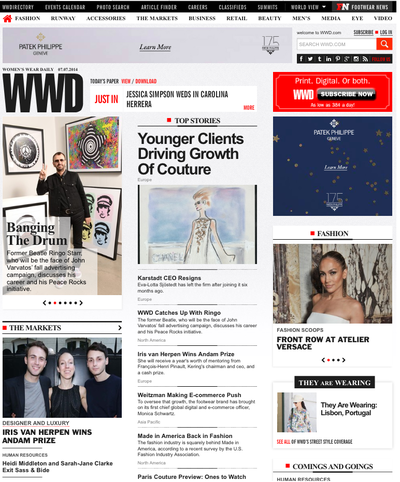A high-resolution screenshot of an online newspaper or magazine, titled "WWD," showcases a variety of engaging content. At the top of the screen, a thin black navigation bar features menu options, followed by a white navigation bar with categories in black text including "Fashion," "Runway," "Accessories," "The Markets," "Business," "Retail," "Reality," "Men's," "Media," "Eye," and "Video."

Prominently displayed, a gray advertisement for Patek Philippe with a "Learn More" link catches the reader's eye. To the left, in bold black capital letters, the magazine's title "WWD" is clearly visible.

Below the title, a captivating image features Ringo Starr standing in an art gallery, surrounded by vibrant, 60s-inspired paintings and illustrations. The caption below, "Begging the Drum," reveals that the former Beatle will be the face of John Varvatos’ fall advertising campaign, discusses his career, and highlights his "Peace Rocks" initiative.

On the right side, a headline reads, "Younger Clients Driving Growth of Couture," accompanied by an elegant watercolor sketch of a woman in a white dress. In the bottom right corner, an image of Jennifer Lopez adds a fashionable touch to the layout.